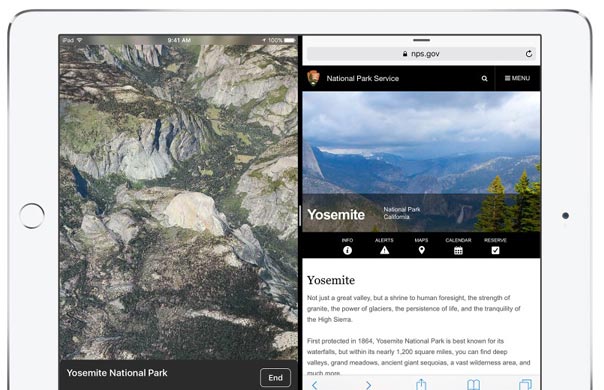The image features a white iPad, a tablet device from Apple Inc., a tech company known for its innovations in mobile phone technology and related services. The iPad screen is split into two sections. On the right side of the screen, a web browser is open displaying the National Park Service (nps.gov) website, specifically focusing on Yosemite National Park in California. The visible webpage provides detailed information about Yosemite, including its history. On the left side of the screen, there's a vivid photograph showcasing Yosemite National Park's majestic mountain range, flourishing vegetation, and the pristine lakes and rivers that traverse the area.